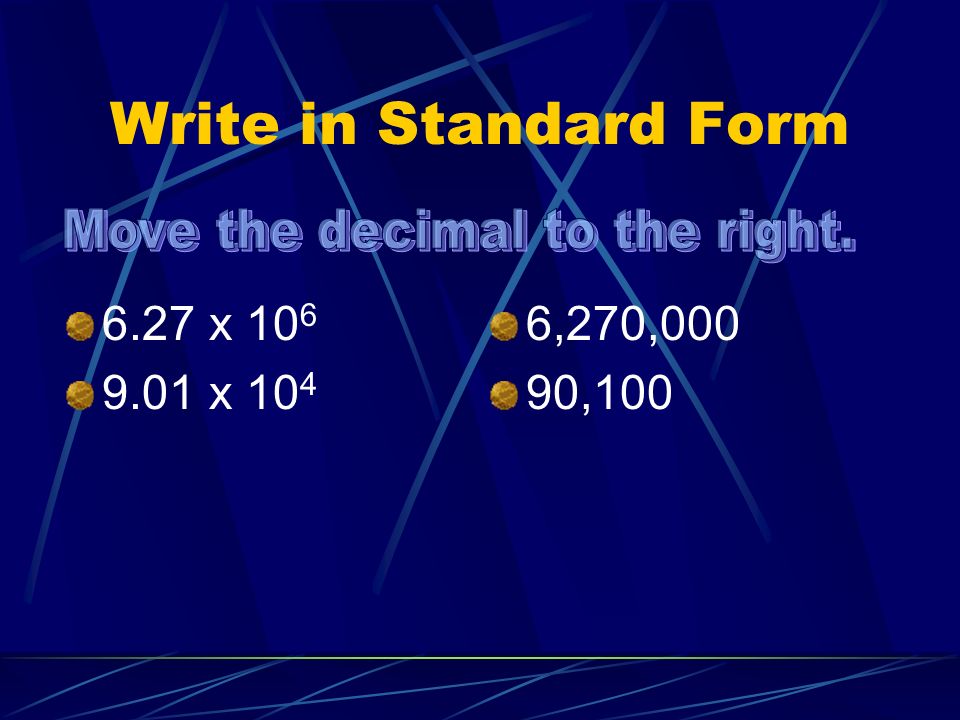The image features a visually engaging blue background with varying shades and a pattern of thin, criss-crossing lines resembling an X-shaped fence. Dominantly displayed at the top in prominent yellow font, the text reads, "Write in Standard Form," with capitalized "W," "S," and "F." Directly beneath, written in light blue, is the instructional sentence, "Move the decimal to the right."

Organized in four bullet points marked by yellow dots, the main content presents a series of mathematical expressions. The first bullet point displays "6.27 × 10⁶," followed by "6,270,000" to its right. The subsequent bullet point features "9.01 × 10⁴" with "90,100" to its right. These numerical representations are presented in white font, emphasizing clarity and aiding comprehension.